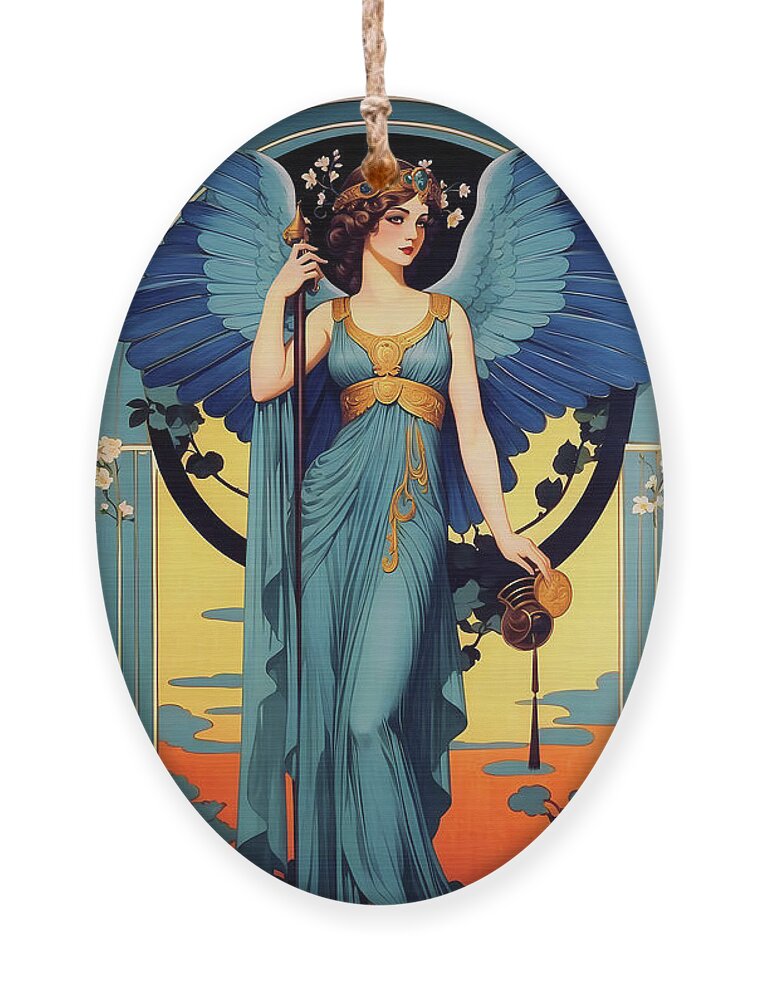The image features an oval-shaped pendant, suspended from a realistic tan rope. Encased within the pendant is an intricately detailed illustration of an angelic woman, capturing a modernized stained-glass art style. The woman, adorned in a flowing turquoise and gold dress that exudes a Greek goddess aura, boasts medium-length dark brown curly hair. She is crowned with a regal headpiece featuring a prominent blue sapphire at its center.

Her majestic wings, a gradient of turquoise and blue, complement her attire. She holds a long golden staff in her right hand, its top embellished with an ornate decorative piece, while her left hand clutches a golden coin. Surrounding her in the background are wisps of clouds, a scattering of delicate white flowers, and vibrant hues of yellow, blue, and orange, evoking a painted sky. This meticulous illustration, set against the pendant's boundary, creates a harmonious blend of realism and artistic fantasy.